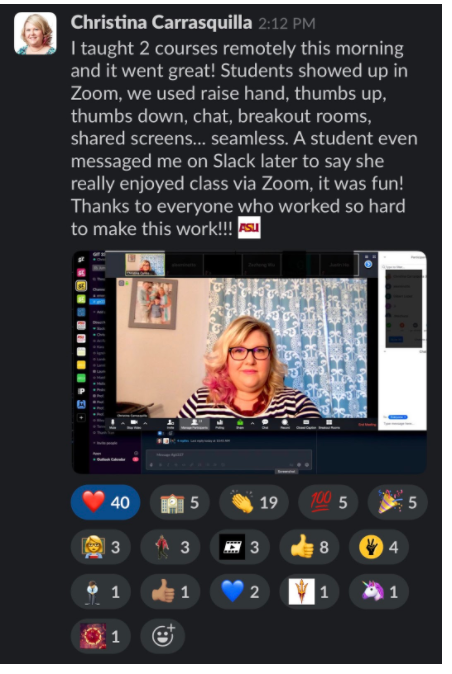**Detailed Caption:**

On this image, it’s a post by Christina Karasquilia. The background is solid black, and Christina's profile icon features a female wearing a blue dress against a white backdrop. The message is written in black text and was posted at 2.12 PM. 

The text reads:
"*I taught two courses remotely this morning and it went great. Students showed up on Zoom. We used raised hand, thumbs up, thumbs down, chat, breakout rooms, shared screen – seamless. A student even messaged me on Slack later to say she really enjoyed the class via Zoom. It was fine. Thanks to everyone who worked so hard to make this work. Asu.*"

The word "Asu" is displayed in red within a white square, acting as an emoji. 

At the center of the image, there is a user interface of a Zoom meeting with Christina teaching. She is dressed in black and white, with a blue-and-white curtain and a world map in the background.

The post includes several reaction emojis at the bottom: 
- Heart (40 likes) 
- Buildings (5 likes) 
- Clapping hands (19 likes) 
- 100 (5 likes) 
- Confetti (5 likes) 
- Teaching (3 likes) 
- Dancing (3 likes) 
- Video (3 likes) 
- Thumbs up (3 different reactions: 8 likes, 4 likes, 1 brown thumbs up) 
- Blue hearts (2 likes) 
- Unicorn (1 like).

This detailed view showcases Christina's successful remote teaching session and the positive engagement from her students and followers.